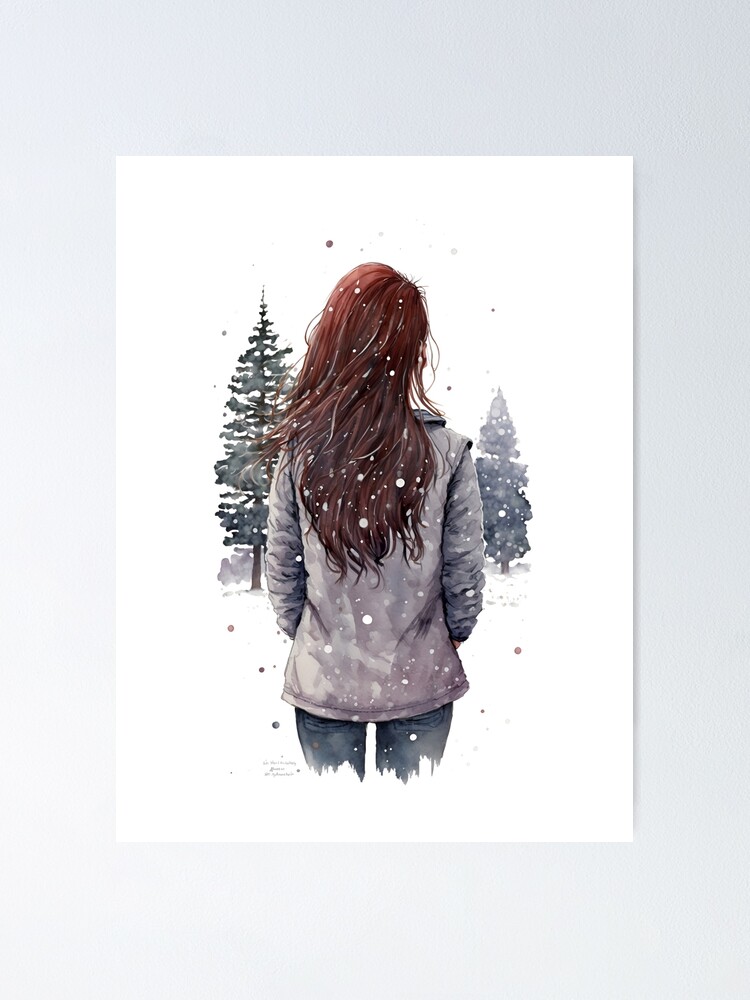The image is a vertically oriented print featuring a central white rectangle on a gray background. Within the white rectangle, there is detailed artwork of a woman viewed from behind. She has long hair, either red or brown, and is wearing a gray coat and dark blue jeans. The woman stands facing two evergreen trees, one on either side of her, against a snow-dotted backdrop. The tree on the right appears slightly faded, possibly due to the depiction of snow. Snow is indicated by both white and darker dots scattered throughout the image. The scene suggests a wintry setting with snowfall and the ground covered in snow. The print is autographed at the bottom left near the woman's leg, though the signature is difficult to read. This print appears to be set against a gray background, perhaps framed or displayed in some manner.